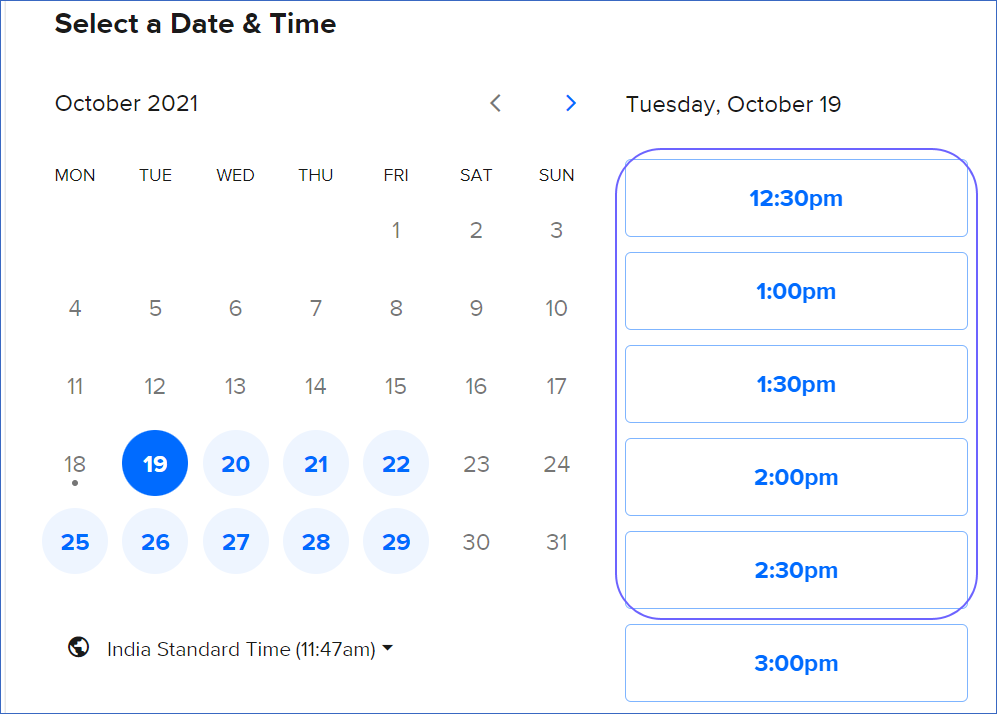The image depicts a screenshot of a Calendly scheduling interface, commonly used for booking meetings or appointments. On the left side of the screen is a calendar for October 2021. At the top, the heading "Selected Date and Time" appears in bold, followed by "October 2021." The calendar highlights the 18th, indicating the current date, and shows available slots for the 19th through the 22nd, with the weekend dates grayed out. Availability continues from the 25th to the 29th.

The date 19th is selected, highlighted by a bolded text. On the right side, detailed time slots for Tuesday, October 19th, are displayed. The time slots are shown in blue rectangular blocks, listed as follows: 12:30 p.m., 1:00 p.m., 1:30 p.m., 2:00 p.m., 2:30 p.m., and 3:00 p.m. Notably, a darker blue rectangle spans from 12:30 p.m. to 2:30 p.m., indicating a reserved or selected timeslot. The 3:00 p.m. slot stands separately, not included within the darker blue rectangle.

Below the calendar, at the bottom left corner, a globe icon is displayed next to the text "India Standard Time, 11:47 a.m." This indicates that the Calendly account is set to India Standard Time, suggesting that the user is based in India.